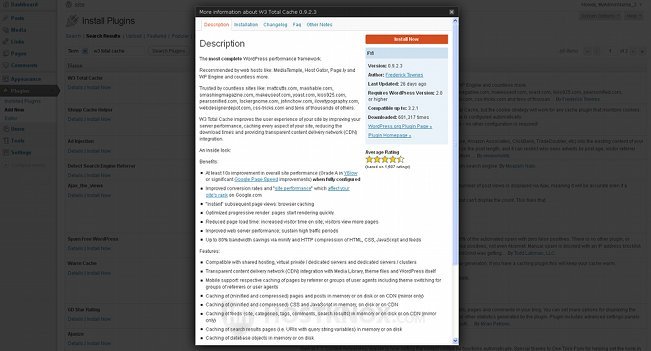The image features a webpage with a white background and predominantly black text, interspersed with some blue text. The main content is small and slightly blurred, making it difficult to read. In the top left corner, there is a clear header that says "Install Plugins." 

Overlaying the webpage is a pop-up notification in the foreground. At the top of the pop-up, it mentions "More Information about WE3: Total Catch." Below this header, there are several tabs, though they are also blurry. The word "Description" is prominently featured. On the top right corner of the pop-up, there is an orange "Install Now" button. 

To the right side of the pop-up, there is a section showing the app's rating, which is an average of 4.5 stars. It is also noted that the app was last updated 28 days ago. Overall, the text throughout the image is small and blurry, making most details difficult to discern clearly amidst the white background and black text.